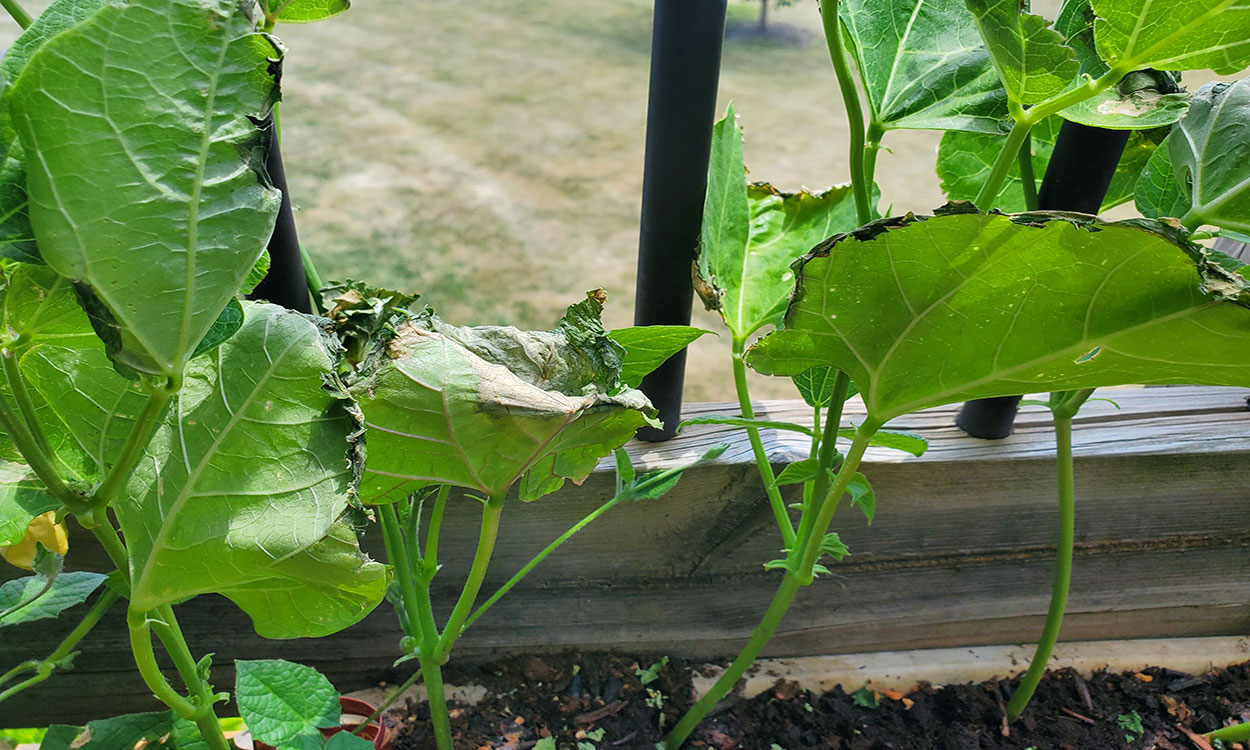In this close-up image, various green plants with a range of leaf shapes are sprouting from rich brown soil. The leaves are detailed enough that their veins and stems are clearly visible. Some of the leaves appear wilted or partially eaten, with dark edges, while others are more full and vibrant. Above the plants, there is a wooden beam with a noticeable horizontal crack, which seems to be part of a balcony. Three black metal bars extend upwards from the wooden beam, suggesting that the garden might be on an elevated or second-floor balcony. In the background, you can see a field with patches of green and brown grass, along with a tree trunk surrounded by its own plot of dirt. The overall scene suggests a sunny day in a natural setting.